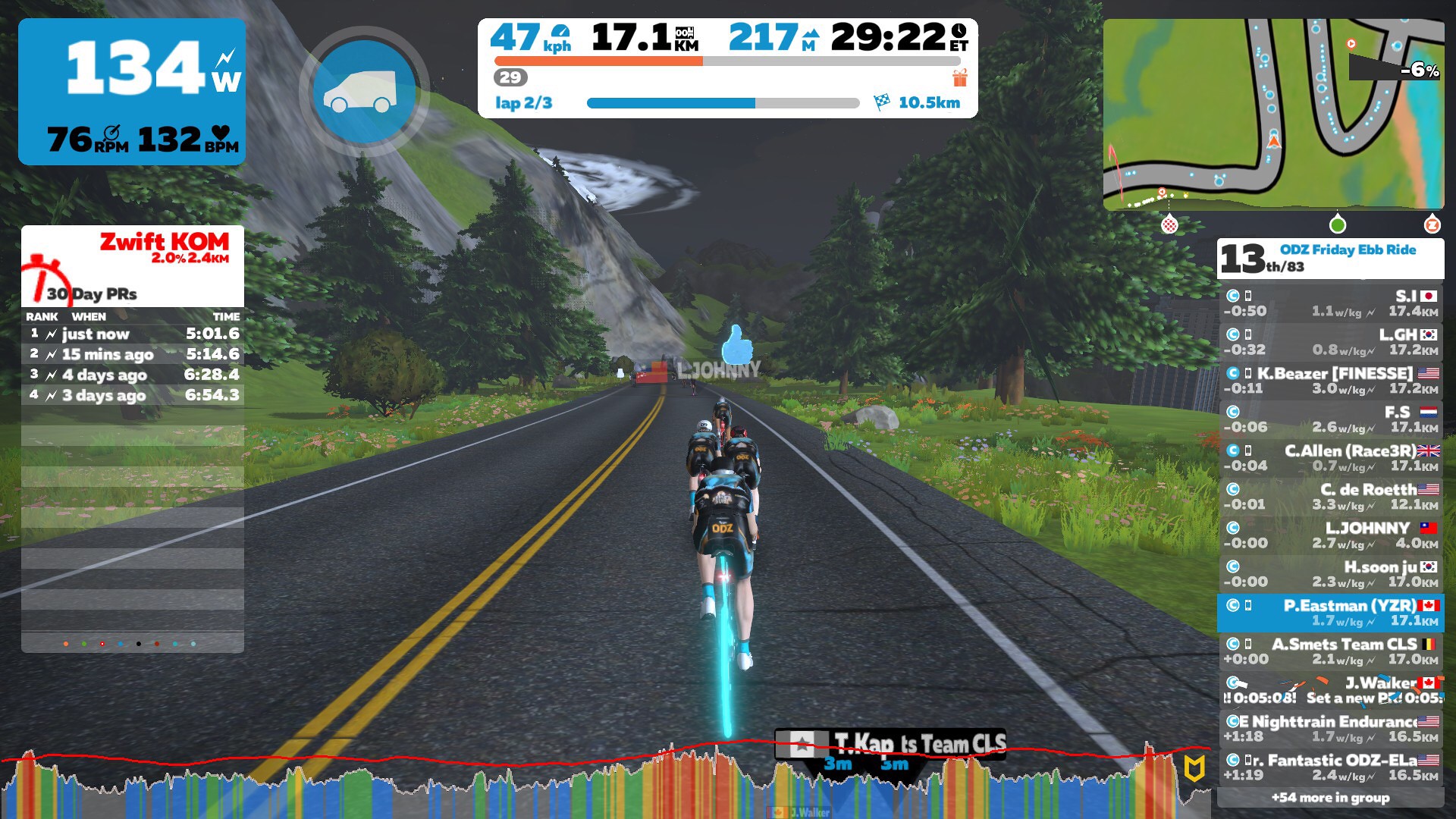This image is a detailed screenshot from a cycling video game, possibly a simulation like Zwift. The scene, rendered in 3D computer graphics, shows multiple cyclists racing away from the viewer on a two-lane gray asphalt road, prominently featuring double yellow lines in the middle and white lines on the shoulders. The road is flanked by fields of vibrant green grass dotted with trees, adorned with lush green leaves. In the distant background, gray cliffs or a mountainside frame the horizon, adding to the scenic landscape.

The game interface is densely packed with various UI elements. In the top right corner, a mini-map showcases a green grassy area with a road bordered by black lines, aligning with the on-screen road. Alongside the mini-map, detailed player stats are displayed, including metrics like wattage (134 W), RPM (76), and heart rate (132 BPM), hinting that the rider is on an exercise machine. The top left section shows more metrics, possibly related to performance and personal records (PRs). Meanwhile, the bottom of the screen features a color-coded wave pattern, likely monitoring exertion levels with red, orange, yellow, green, and blue hotspots. Additionally, there is a scoreboard on the right side listing participants and their current statuses.

The cyclists themselves are depicted with bicycles outlined in neon blue lights, with the player’s own back tire glowing a striking cyan color, adding a futuristic touch to the setting. The vibrant environment and comprehensive interface suggest an immersive and interactive cycling experience, blending real-time data and virtual visuals seamlessly.